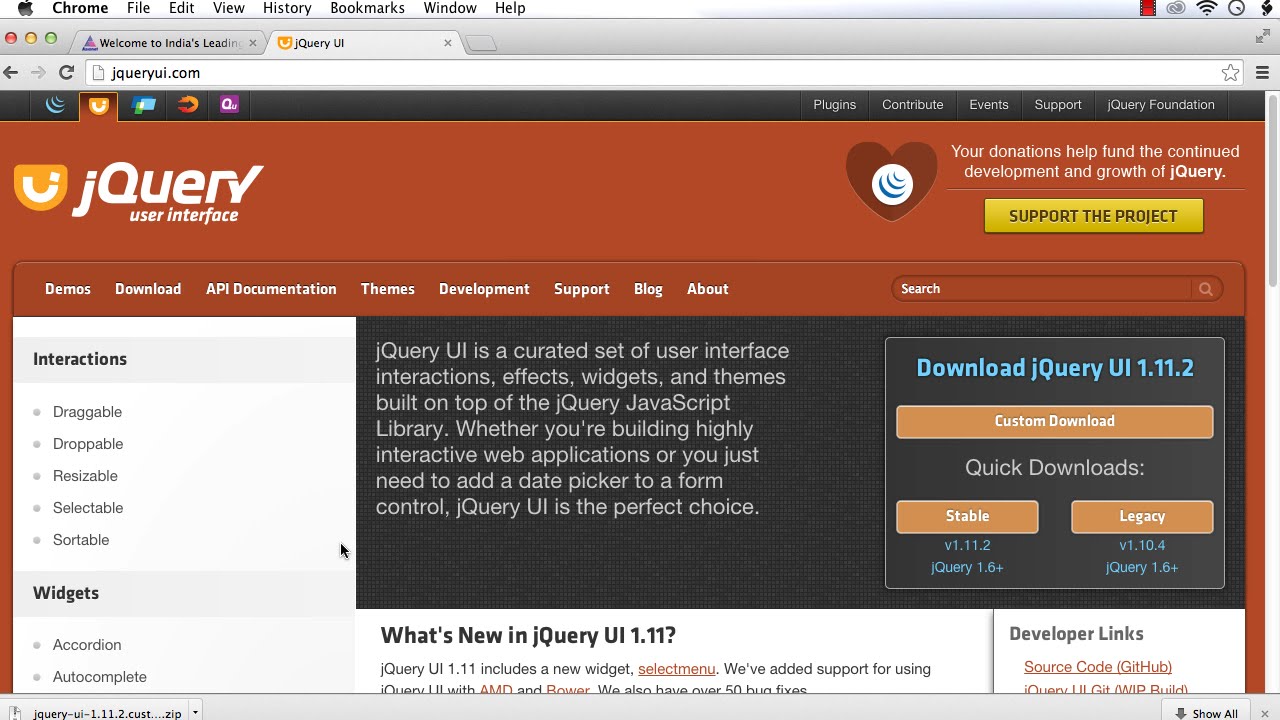In this detailed image, we're viewing a Mac computer screen, identified by the distinctive Apple logo with a bite taken out of it in the top left corner. The menu bar reads "Chrome, File, Edit, View, History, Bookmarks, Window, and Help," with "Chrome" being highlighted in black, indicating that it has focus. Moving rightward, the bar features a film icon, a linked chain icon, the Wi-Fi signal icon displaying connectivity, a clock, and a plug icon on the far end.

Beneath this bar is a gray strip housing two tabs. The first tab, titled "Welcome to India's Leading," is a dark gray and marked with a small 'x' for closing. Next to it are the three Mac traffic lights – red, yellow, and green. Adjacent to this is a tab labeled "jQuery UI," exhibiting a logo resembling a jumbled 'J' on its side against an orange half-oval background, also with a closing 'x'.

To the right end of this bar are double arrows, pointing northeast and southwest. Below, a lighter gray navigation bar has a back arrow, a forward arrow (grayed out), a refresh button, a URL field showing "jQueryUI.com," a page icon with a folded corner, a star bookmark icon, and a "settings" icon represented by three stacked lines.

The main screen has a black background. Its focal point is the jQuery UI website, with an orange and white theme. The central image contains three concentric curved lines, shrinking in size from the largest to the smallest, right above the jQuery icon, indicating focus on this tab.

Several icons on the screen are less identifiable. They include a blue rectangle with a green piece and a yellow rectangle inside, an orange icon with a right-pointing arrow, and a purple square with "QU" inscribed. To the extreme right, the navigation menu lists "Plugins, Contribute, Events, Support, and jQuery Foundation."

The jQuery main content area is rust-colored with a black segment framed in white. Prominently displayed is a heart with three blue converging lines saying, "Your donation helps fund the continued development and growth of jQuery." Below, a mustard-colored Support the Project button in black, uppercase letters catches the eye.

Further down, a navigation menu appears with links such as "Demos, Download, API Documentation, Themes, Development, Support, Blog, About," all in a darker rust hue. Search functionality is offered via a light rust-colored bar bearing a magnifying glass icon.

On the left pane, which is entirely white, two headers—"Interactions" and "Widgets"—stand out in bold. Under Interactions are five options: draggable, droppable, resizable, selectable, and sortable. Widgets feature two bullet points: accordion and autocomplete.

The central black pane with white text describes jQuery UI as an enhanced set of user interface elements built atop the jQuery JavaScript library, suitable for interactive web applications or simple additions like date pickers. There’s a link to "Download jQuery UI 1.11.2" in blue.

Three buttons follow. An orange "Custom Download" button with white text, and beneath the gray Quick Downloads header, two more buttons: the white-on-orange "Stable" for version 1.11.2 and the orange-on-white "Legacy" for version 1.10.4. 

Blurbs at the bottom highlight updates—"What’s new in jQuery UI 1.11" explains additions like the Select Menu widget, AMD, and Bower support along with 50+ bug fixes. 

Lastly, a developer links section includes references to Source Code on GitHub and jQuery UI Git WIP Build. At the very bottom, a box displays "jQuery-ui-1.11.2.cust..." with a "Show All" button and a closing 'x' icon.